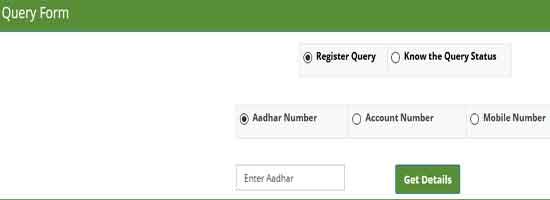The screenshot depicts a query form on a website, accessed on a device with a landscape orientation, likely a laptop, desktop computer, or tablet. The top section features a green navigation bar with white text reading "Query Form." Directly below this bar are two selectable options: "Register Query" and "Know the Query Status," with "Register Query" currently selected.

The form provides three identification options: Aadhaar Number, Account Number, and Mobile Number, with "Aadhaar Number" (spelled A-A-D-H-A-R) selected by default. Below this selection, there's an empty text box labeled "Enter Aadhaar," designed for users to input their Aadhaar Number. A green button labeled "Get Details" is situated beneath the text box. A thin green line, matching the top bar and button, appears at the bottom of the screen segment, maintaining the page’s cohesive color scheme.